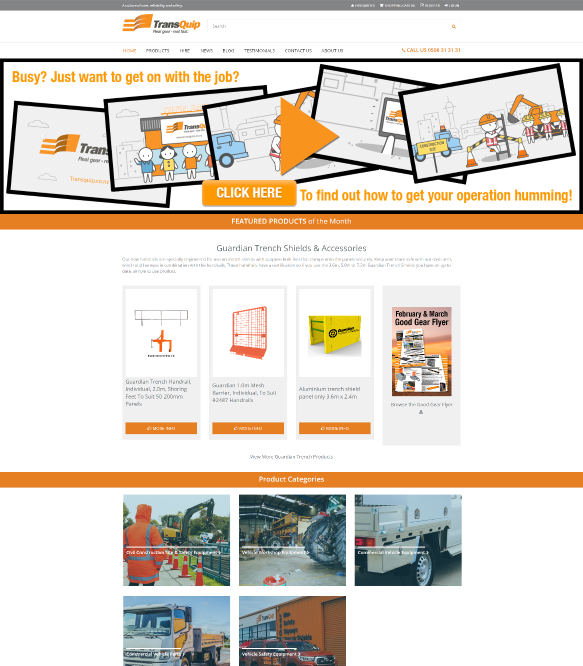Screenshot of TransQuip Website: The top of the page features the company's flag-like logo alongside the name "TransQuip" in bold black and orange lettering. Below the logo, a white navigation menu is visible, though the categories are too small to decipher. Centered on the page is a clickable video with an accompanying button labeled "Click here to find out how to get your operation going." Beneath the video, there are four distinct categories of equipment prominently displayed. At the bottom of the page, five images showcase trucks, vehicles, and heavy machinery, each with text superimposed on top, likely serving as links, though the text is too small to read.